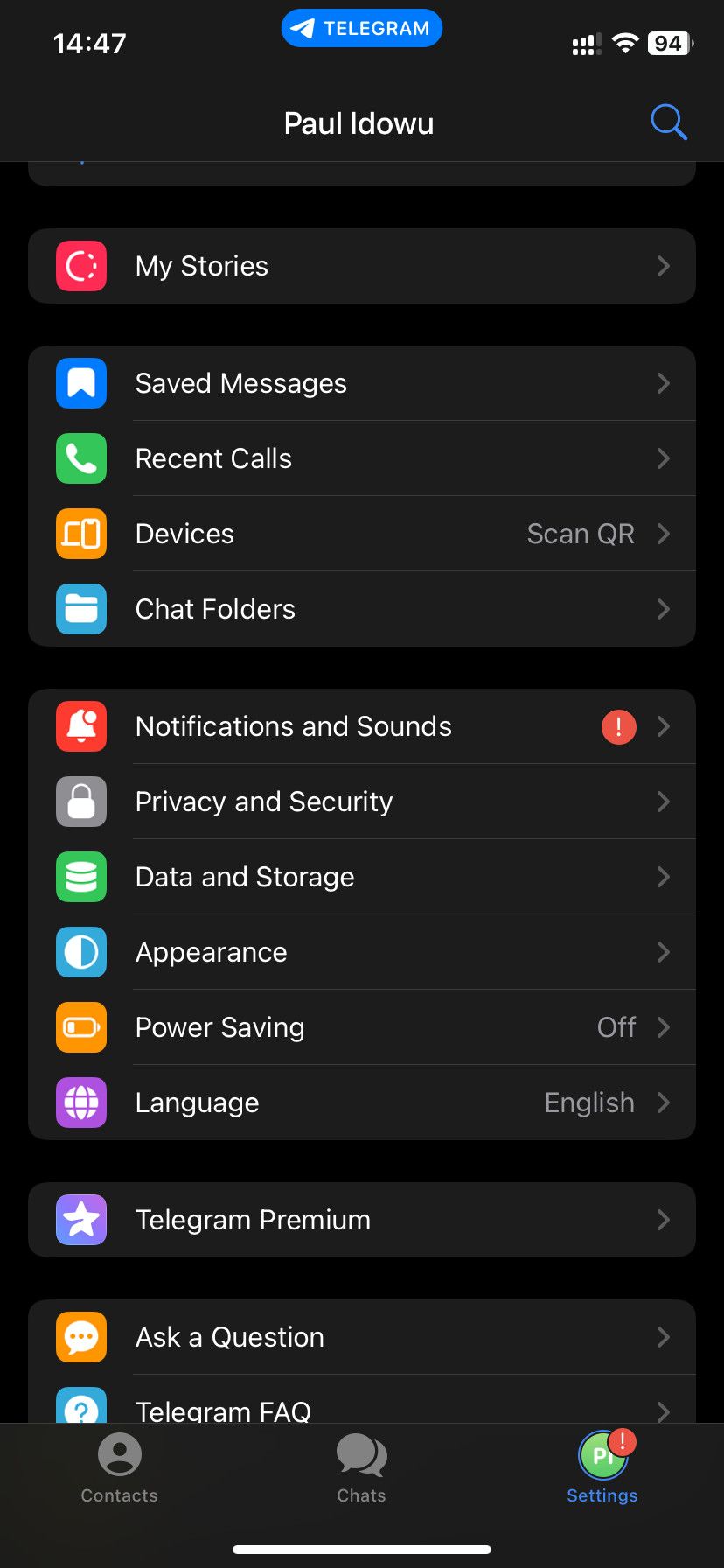This is an image of a cell phone screen displaying the Telegram app interface against a black background. The top left corner of the screen shows the time as 14:47, while the top right corner indicates a battery life of 94%. In the center of the screen, there's a prominent blue button featuring the Telegram logo, a white paper airplane on a blue background. The user appears to have selected a contact named "PAW Idowu," with the name displayed in white text. Below the name, the option "My Stories" is visible.

Running vertically down the left side of the screen are several colorful icons, each accompanied by explanatory text. The list begins with a reddish square labeled "My Stories," followed by a blue icon for "Saved Messages," a green icon for "Recent Calls," and an orange icon labeled "Devices." Light blue is used for "Chat Folders," followed by a red bell icon labeled "Notifications and Sounds." Adjacent to this red bell icon, towards the right edge of the screen, there's an exclamation mark encircled in red. The list continues downward in the same manner, indicating various features and sections within the app.